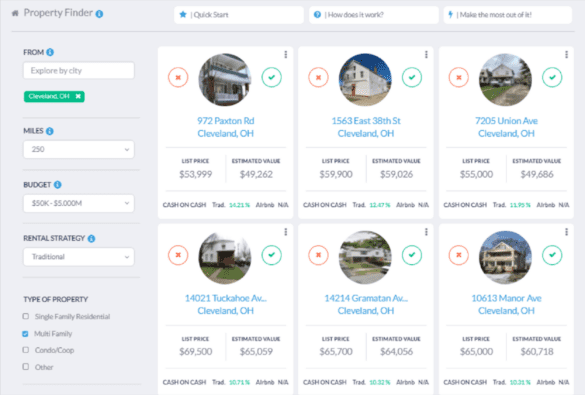In the emergency property finder interface, the left pane displays a search field refined by city, showing properties up to 250 miles away within a price range of $50,000 to $5,000,000. The search focuses on traditional rental strategies and includes various property types such as multifamily, single-family residential, condos, co-ops, and others, with multifamily currently selected. Three property options are highlighted:

1. 972 Paxton Road, Cleveland, Ohio: Listed at $53,999 with an estimated value of $49,262.
2. 1563 East 38th Street, Cleveland, Ohio: Listed at $59,900 with an estimated value of $59,026.
3. 7205 Union Avenue, Cleveland, Ohio: Listed at $55,000 with an estimated value of $49,686.